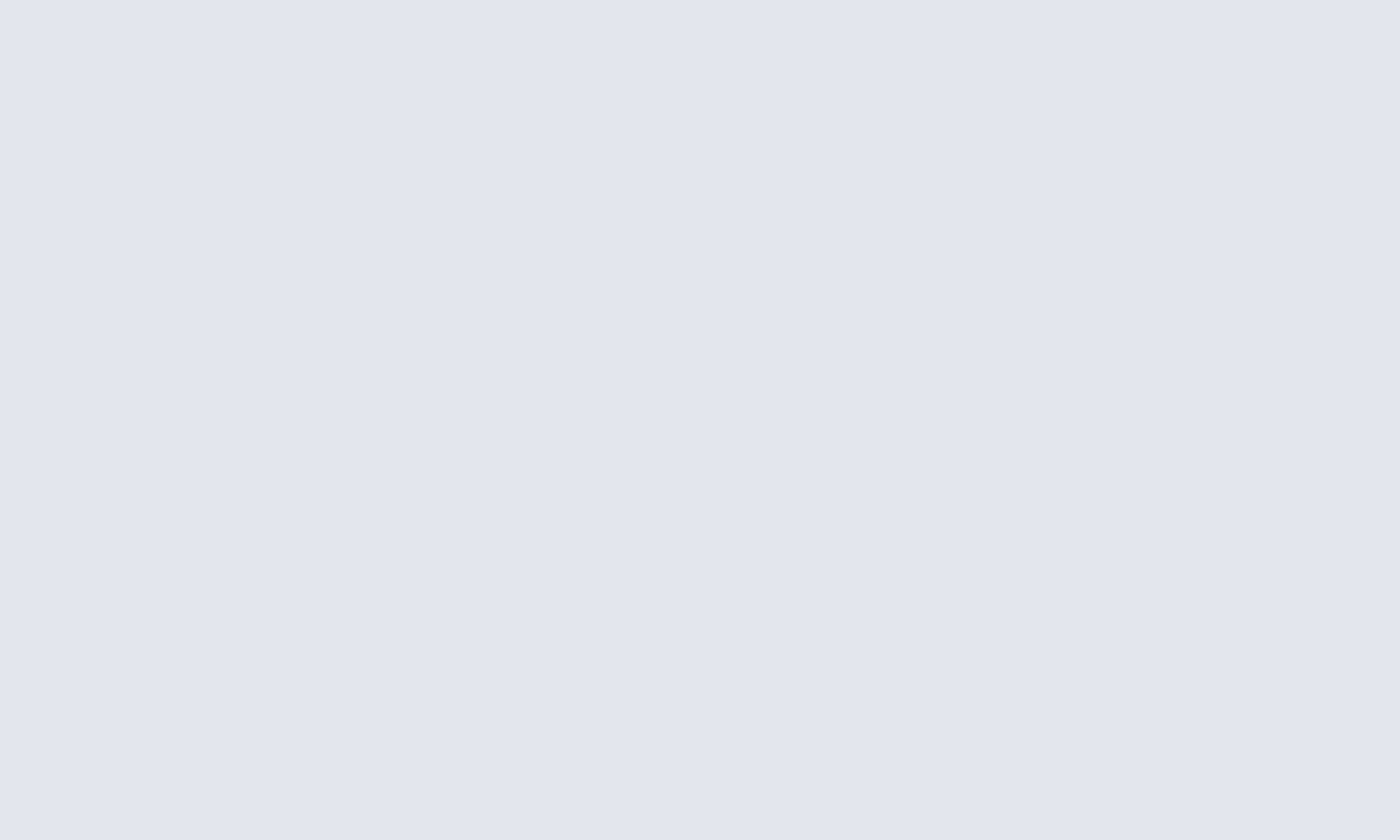A gray surface occupies the entirety of the image, suggesting the potential to represent multiple technological elements. The object appears rectangular, akin to a piece of construction paper in a landscape orientation, but given the context of technology, it is more likely indicative of a blank computer screen. This screen might be powered off or in sleep mode, contributing to its featureless appearance. Another plausible interpretation is that the image shows the backside of a laptop lid, potentially from an older MacBook Air or similar device devoid of branding or logo. Intriguingly, the uniform grayness could also be an artistic representation, possibly a child's minimalist drawing of a computer. The surface lacks any form of distinguishable content—no icons, text, or symbols interrupt the slate-like monotony, and it contributes no detail to suggest depth, texture, or interaction, leaving viewers to ponder its true nature.